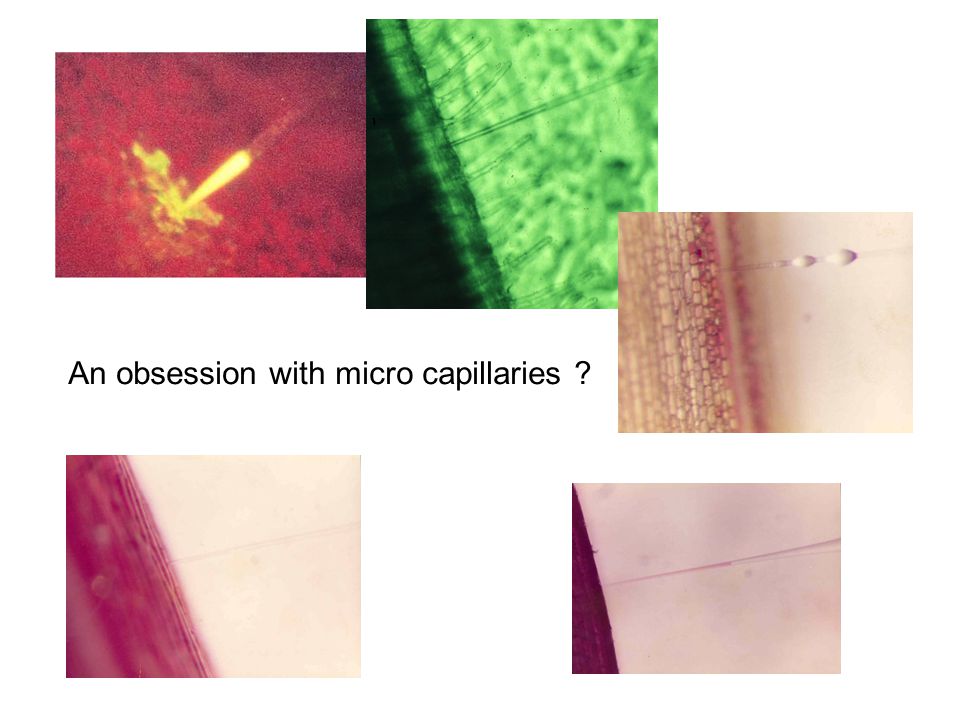A collage of five microscopic images, arranged with three on top and two on the bottom, surrounds a central text that reads, "An obsession with micro capillaries?" in small, black, sans serif font on a white background. The images, presumed to depict microscopic views of micro capillaries, feature themes of needles piercing skin. Starting from the top left and moving clockwise, the first image is dominated by intense red hues and appears to show a burning needle's yellow tip piercing skin. Next, a green-toned image displays dark green skin on the left transitioning to light green on the right, with visible hairs and a needle moving from right to left across the skin. The top right image has beige skin with red hues, water droplets on a needle moving from left to right across the frame. The bottom left picture, similar in theme, shows red skin on the left against a beige background. Lastly, the bottom right image, the smallest, depicts a deep red section of skin on the left, against a beige background with a needle coming from the right. The overall color scheme of the collage features various shades of red, green, and purple, contributing to an intense, almost clinical aesthetic.